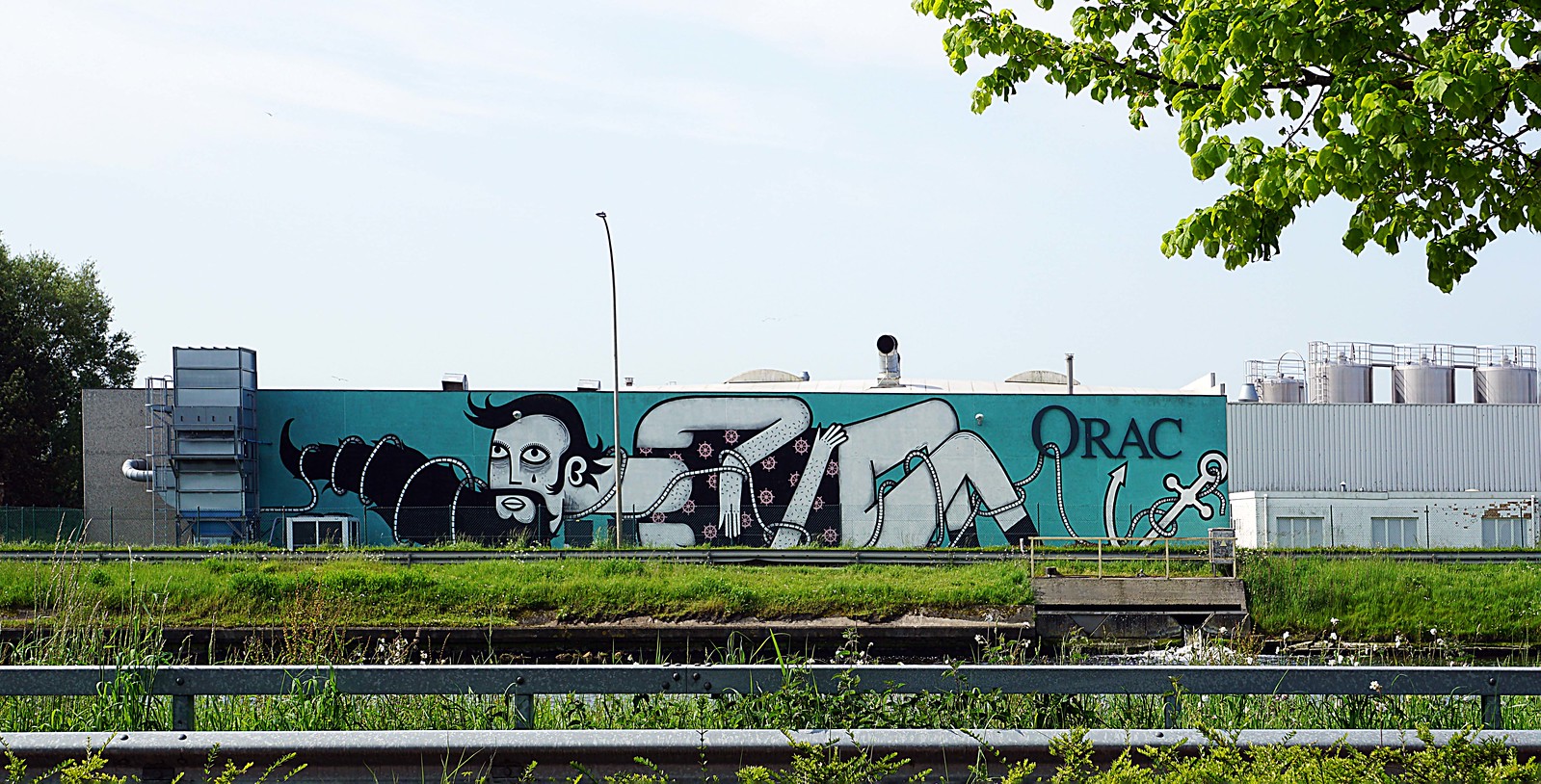In the foreground of the image, a double metal rail set into the ground with metal posts lines the side of a road, transitioning into an area that appears to be train tracks. An elevated section of land, supported by stone and concrete retaining walls, rises beyond this point, featuring more metal railings possibly for an additional road or tracks. Dominating the background is a rectangular, industrial-looking building made of metal with a distinct blue-painted side. The mural adorning this side of the building is surreal and Picasso-esque, depicting a bearded man lying on his side. His elongated neck extends unnaturally to the left, with his head turned in an improbable direction. Wrapped around his legs, arms, and neck is a rope that resembles a pearl necklace, leading down to a white anchor at his feet. The man appears to be wearing a t-shirt with a floral pattern, though the absence of bottoms and any defining feature at his crotch adds to the surreal quality of the artwork. The setting appears to be an open area during daytime, with a clear view of what seems to be additional metal structures, likely part of a factory or industrial complex, to the right of the painted building.